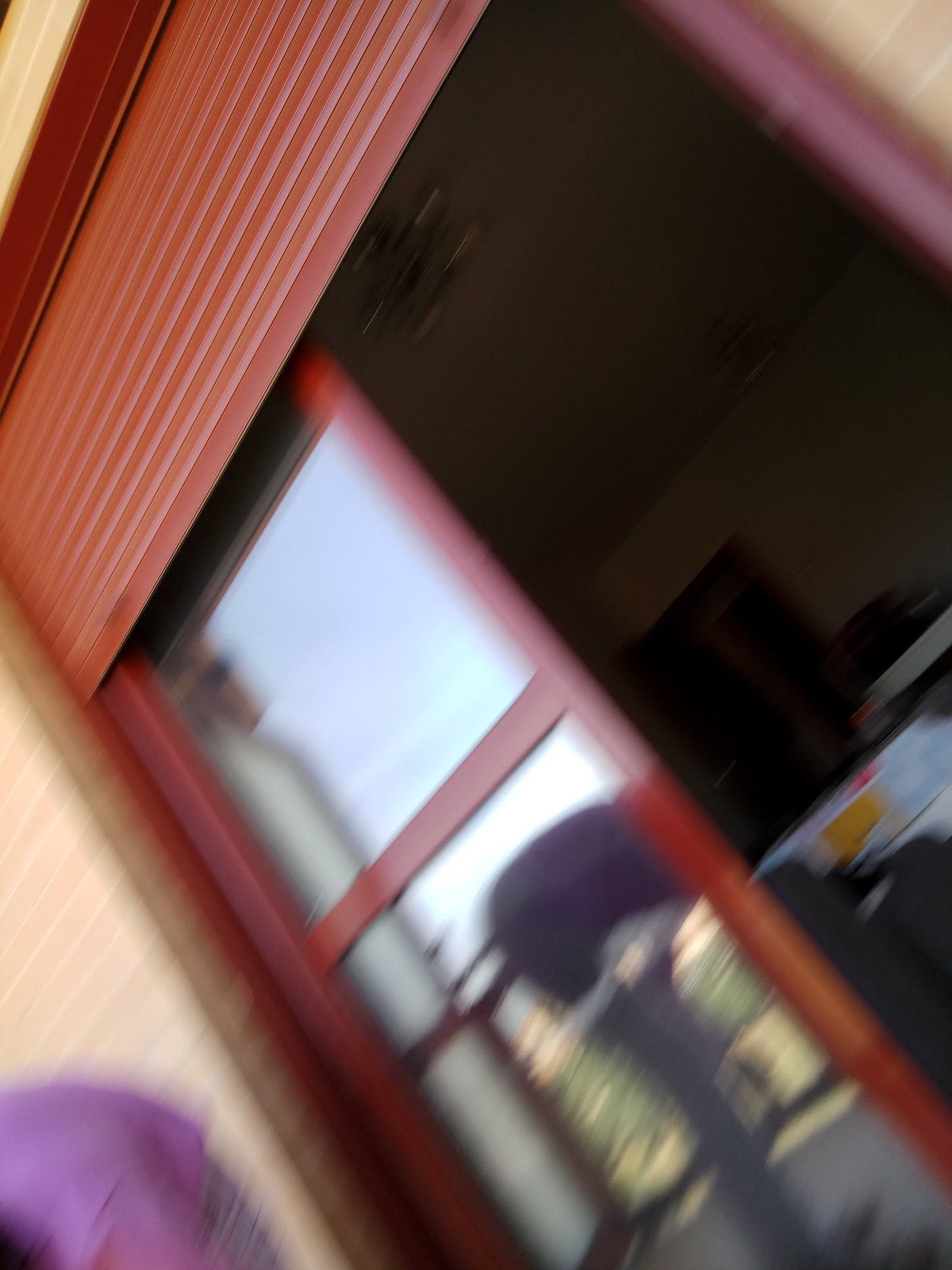This image, albeit blurry, depicts a scene viewed from the outside looking into a room through a set of French doors. The doors are characterized by their red frames and clear glass panes, one door is slightly ajar, and the other is fully open. A light tan brick wall appears to the left of the doorway. Above the doors, there is a red, ridged or louvered header which may be wood or metal, and a rolled-down garage door mechanism that could cover the doors.

The reflection on the closed door shows a glimpse of the outside environment, with hints of blue sky, green grass, and an indistinct object. It also captures the shadowy silhouette of a person in a purple shirt and gray pants, bent over at a 90-degree angle. Inside the room, the lighting is dim, but a white table and another doorway can be discerned. The interior walls are light brown, and there is a silver chandelier hanging from the ceiling, adding to the overall muted ambiance of the space. The image is slightly rotated, giving an odd angle perspective to the viewer.